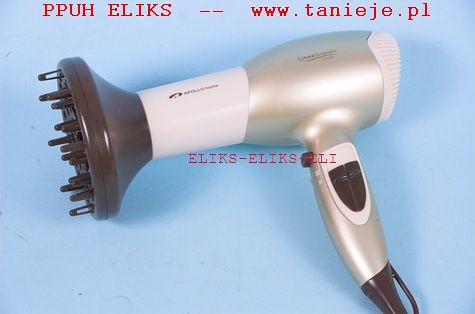This is an up-close color photo of a hair dryer with a brown diffuser attached at the end, designed to prevent curls from getting blown out. The dryer, in the shape of a pistol, features a distinct metallic goldish-silver body with a white middle section and a white nozzle where the hot air is expelled. The handle is also silver and includes brown switch buttons for controls, with a prominent red trigger that likely functions as the cold air button. The cord's connection point and the plastic covering it are brown. The dryer is set against a light blue background, and text in red on the top reads "P-P-U-H E-L-I-K-S--W-W-W.tanieje.pl," followed by "E-L-I-K-S--E-L-I-K-S--E-L-I."